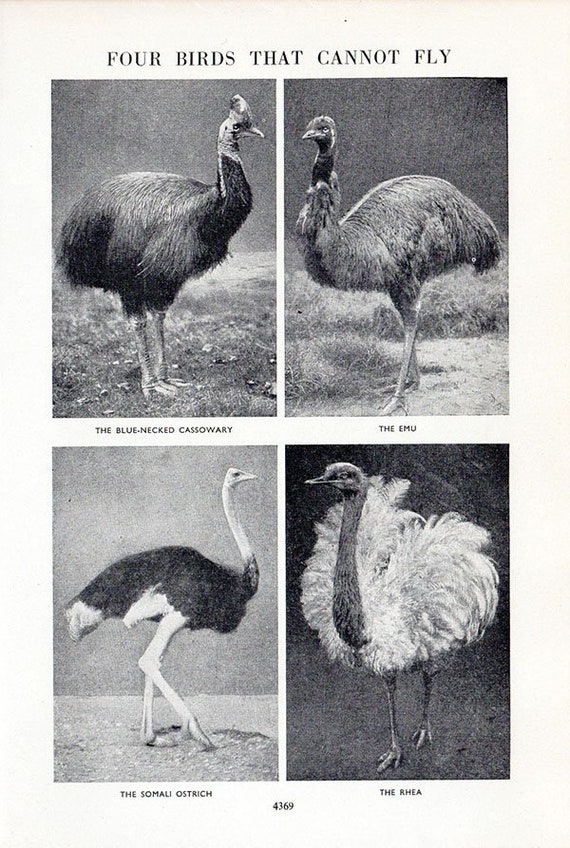This black-and-white photograph showcases four different kinds of flightless birds, arranged in a grid format with two images at the top and two at the bottom, labeled in bold uppercase letters at the top as "FOUR BIRDS THAT CANNOT FLY." The birds featured are the blue-necked cassowary, the emu, the Somali ostrich, and the rhea. Each bird exhibits a strikingly tall stature, with long, powerful legs designed for running. The birds share a general ostrich-like appearance with elongated necks and minimal wing development, except for the rhea which appears more bushy and outwardly expanded, reminiscent of a peacock. Despite the uniform black-and-white coloration, the structural details highlight their majestic and robust physiques, underscoring their adaptation to a terrestrial lifestyle.